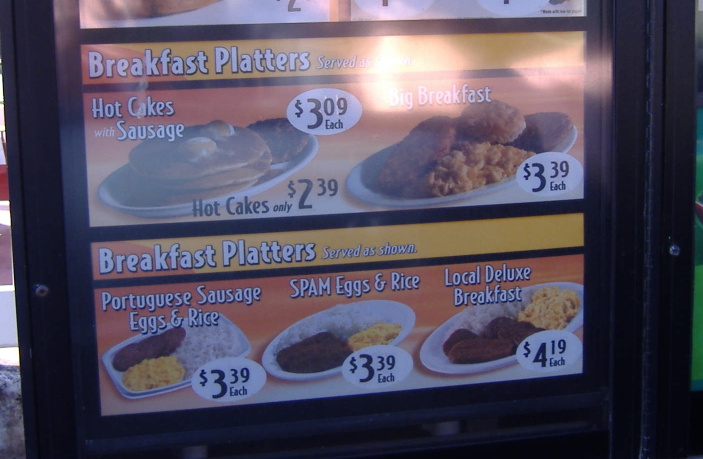The color photograph captures an outdoor scene focusing on a restaurant's menu sign. The menu is encased in a black frame and features vivid pictures of various breakfast items for sale. The sign is positioned on a sidewalk composed of concrete or stone. 

Prominently advertised at the top of the menu are breakfast platters, each accompanied by colorful images to entice customers. One highlighted item is the hotcakes and sausage platter, priced at $3.09. If ordered separately, the hotcakes alone are listed at $2.39. Another featured option is the "Big Breakfast," which includes hash browns, biscuits, eggs, and sausage, available for $3.39.

Below these primary items, several other breakfast platters are showcased: Portuguese sausage, eggs, and rice for $3.39, as well as Spam, eggs, and rice for the same price. Lastly, the menu presents a special offering: the "Local Deluxe Breakfast," an extensive meal featuring additional sausage, rice, eggs, hotcakes, and possibly hash browns, priced at $4.19.